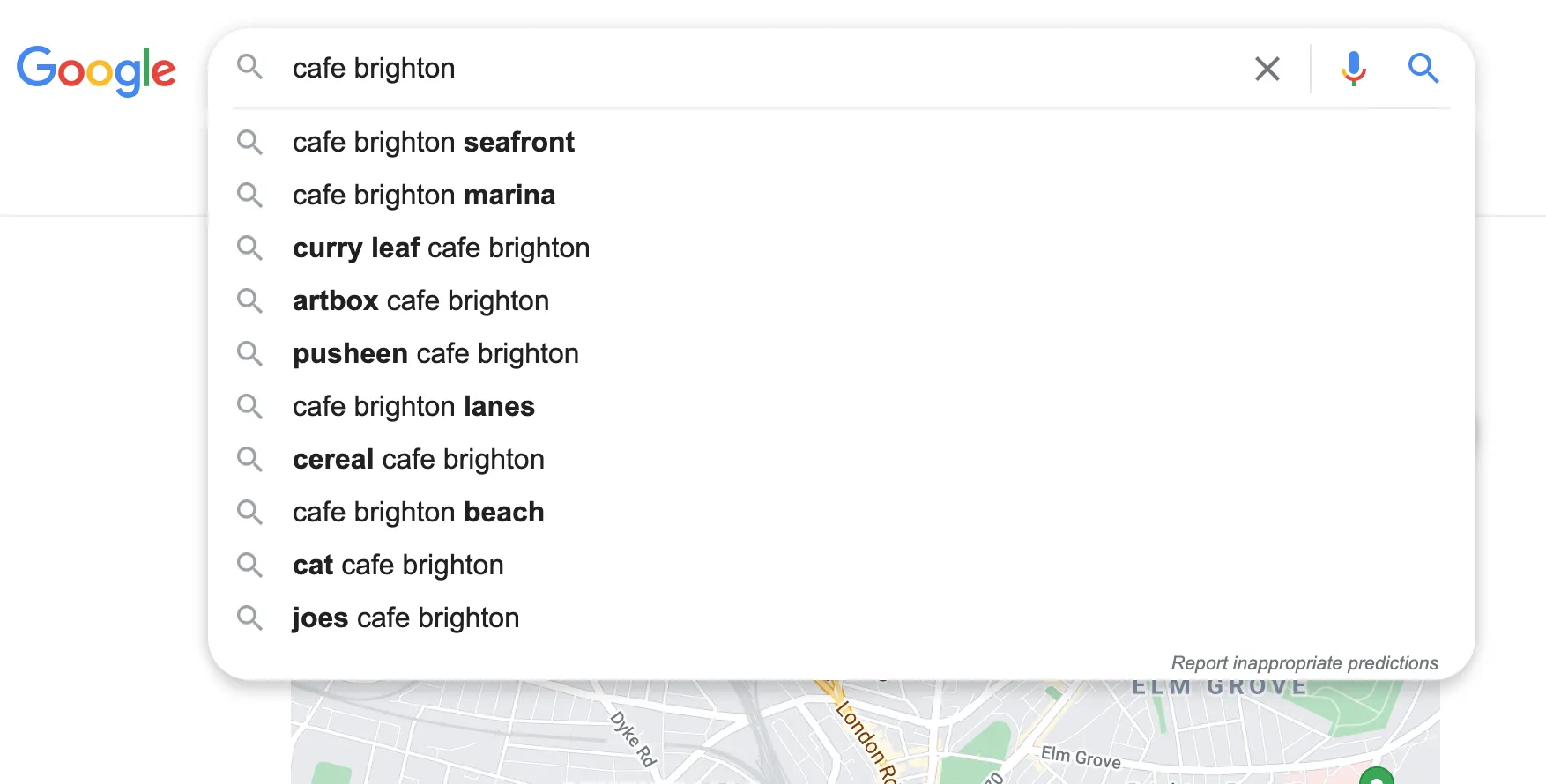The image displays a Google search interface superimposed over the bottom section of a map, which has a gray background with white roads labeled in light gray text and some green spaces visible. In the upper left corner, the colorful Google logo is prominently featured, with a search bar situated to its right. Adjacent to the search bar are a bright blue and red microphone icon and a blue magnifying glass icon.

The search query, "Cafe Brighton," is entered in black text within the search bar. Below the bar, a list of suggested search options provided by Google is shown in a vertical sequence: "Cafe Brighton Seafront," "Cafe Brighton Marina," "Curry Leaf Cafe Brighton," "Art Box Cafe Brighton," "Pusheen Cafe Brighton," "Cafe Brighton Lanes," "Cereal Cafe Brighton," "Cafe Brighton Beach," "Cat Cafe Brighton," and "Joe's Cafe Brighton." For each suggestion, all words except "Cafe Brighton" are highlighted in bold black text, while "Cafe Brighton" remains in regular black text.